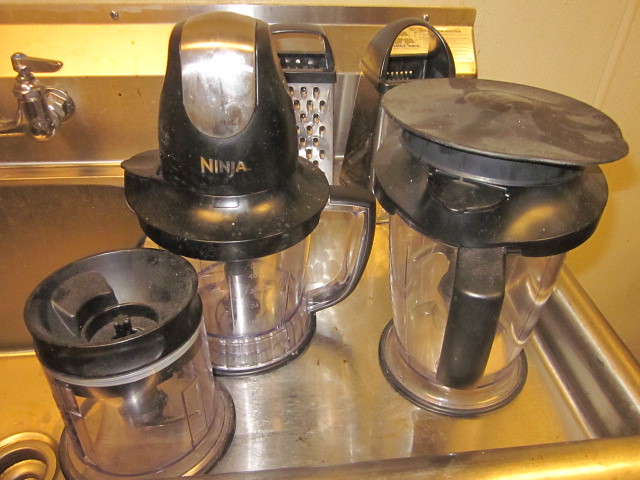This is a detailed color photo depicting a commercial-style stainless steel sink with an integrated counter and drain board. The square basin sink is accompanied by a silver spigot faucet located on the left side. The image prominently features several cooking tools, notably parts of a Ninja food processor and blender set. Central to the arrangement is a clear plastic container with a black handle and lid, branded with "Ninja." To the right is a larger similar container with a lid for storage, along with a smaller counterpart in the foreground. All of these pieces feature central mechanisms indicative of their food processing functionalities. Situated in the background are two upright manual cheese graters with black handles, contributing to the culinary ensemble. The scene is illuminated by a soft, yellowish light, enhancing the industrial ambiance of the stainless steel environment.